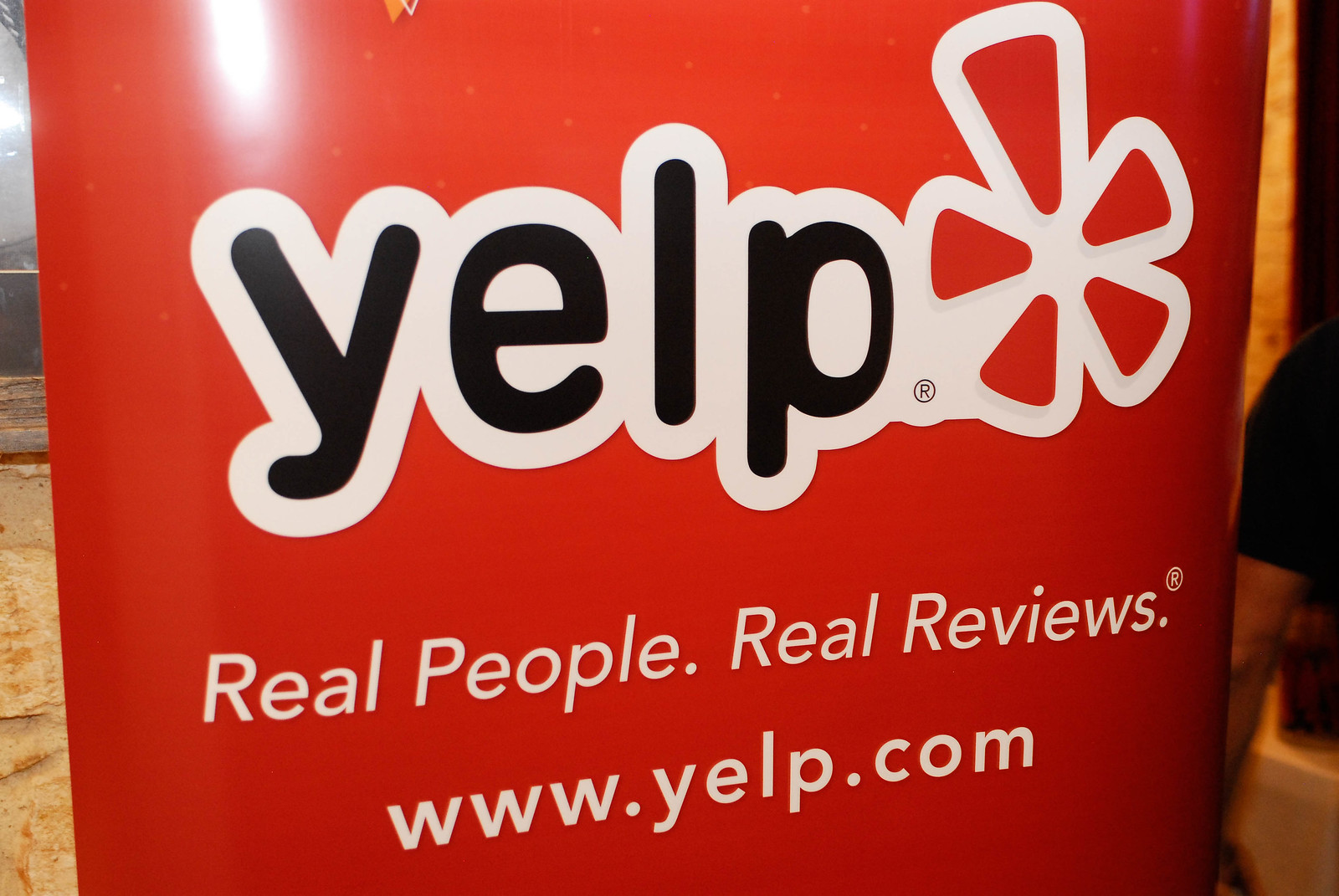The image captures a vibrant red advertisement banner for Yelp, prominently displayed against what appears to be a lobby or office setting. The banner, possibly floor-standing, features the word "Yelp" in bold black font with a distinct white outline, accompanied by the recognizable Yelp logo—a stylized emblem resembling pizza slices. Beside the logo is a registered trademark symbol (®), underlining the official nature of the advertisement.

Below the main branding, the tagline "Real People. Real Reviews." is clearly visible in white font, also accompanied by a registered trademark symbol (®). Further down, the web address "www.yelp.com" is neatly inscribed in white font.

The red background of the sign is glossy, adding to its standout appearance. On the right edge of the photo, part of a man's arm, clad in a black shirt, is visible, giving a sense of scale and human presence. To the left, there's a glimpse of a light brown tiled floor and some overhead lighting, reinforcing the indoor, possibly lobby-like environment.